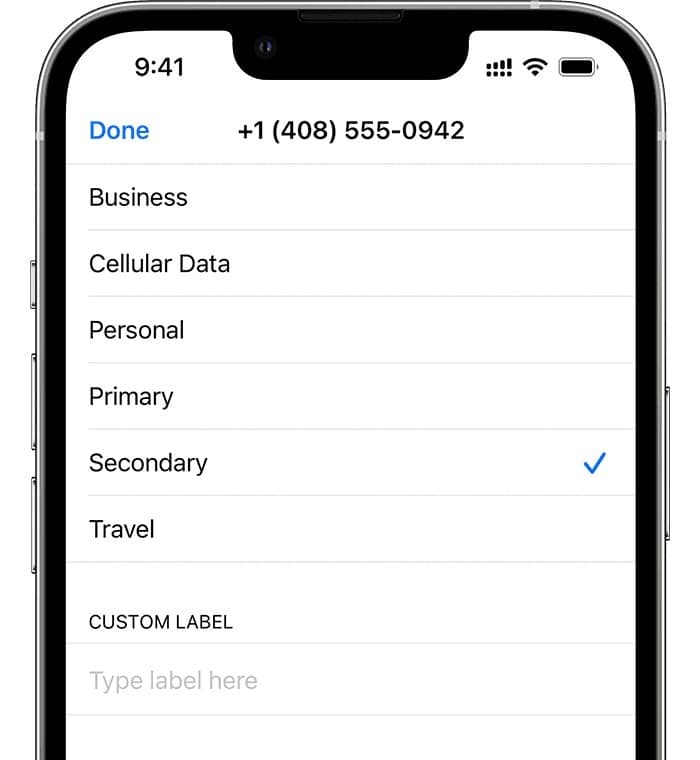In this smartphone screenshot, the interface indicates it is 9:41 AM, as shown at the top of the display. The device has full cellular reception with 4 bars, active Wi-Fi, and a fully charged battery. Beneath the time, the word "Done" is highlighted in blue, and next to it is a contact number displayed as "+1 (408) 555-0942." 

A vertical list of options is presented on the left-hand side of the screen. The options are categorized as follows:
1. Business
2. Cellular Data
3. Personal
4. Primary
5. Secondary (noted to be selected with a blue checkmark)
6. Travel

The background is white, and the dark outline of the smartphone frame is clear, showing the silver casing and side buttons of the device. At the bottom of the page, there are two additional rows: one labeled "Custom Label" and the other prompting "Type Label Here" in a light gray font, indicating text-entry fields.

The image captures a detailed view of the phone's interface, emphasizing the robust organizational features and current settings of the mobile device.